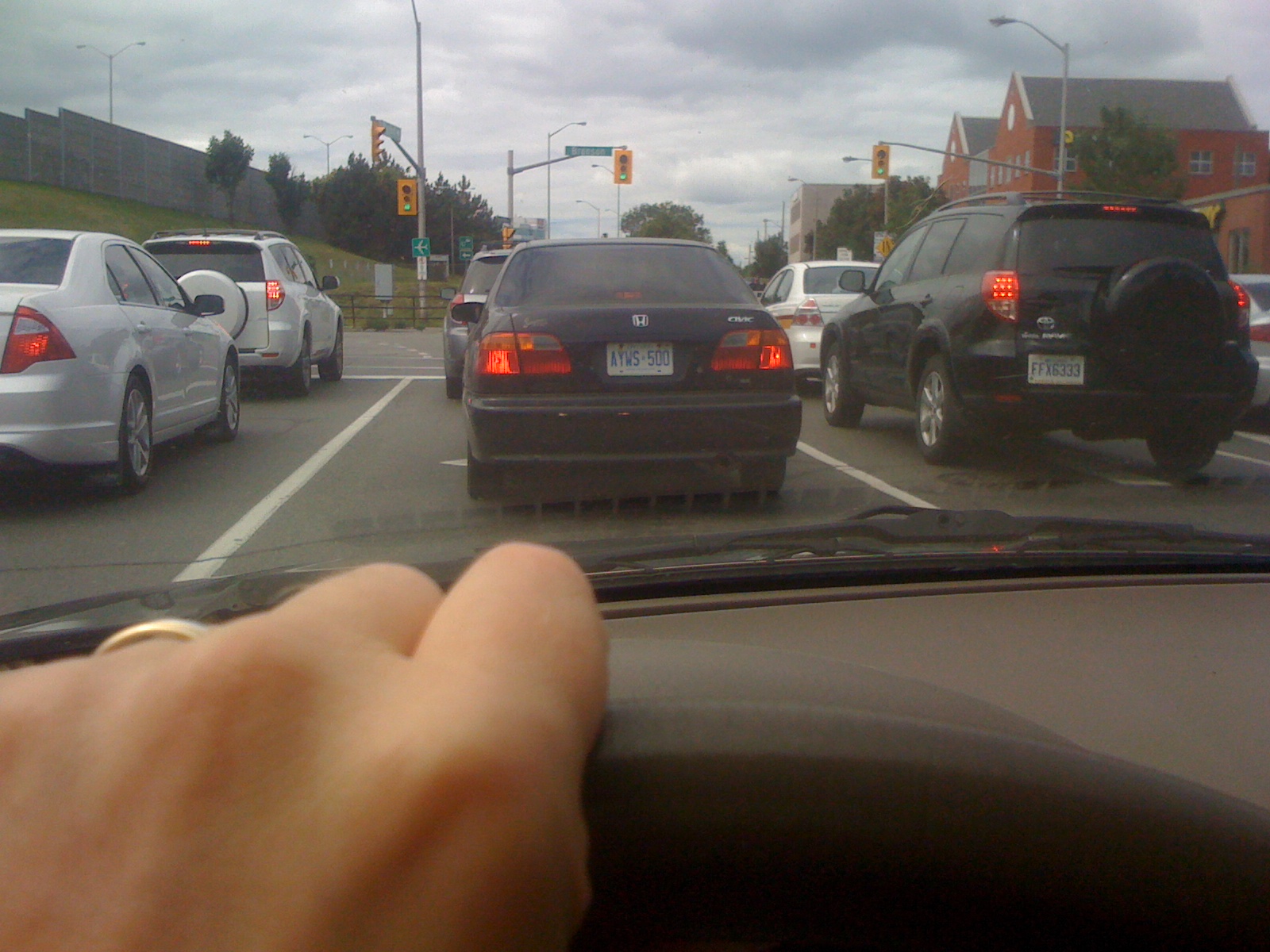The image captures a first-person view from the driver's seat, with the driver's hand, adorned with a ring, gripping the steering wheel at the 12 o'clock position. The scene depicts a green-lit intersection with multiple vehicles ahead. Directly in front of the driver is a steel gray sedan, followed by a black vehicle whose make is indeterminate. To the right of this black vehicle, there is a white Kia, and beside it in the far-right lane, there's another black SUV. Further back, another black sedan can be spotted in front of a white vehicle. On the far left lane, another SUV is visible. Red brick buildings with gray roofs are noticeable in the upper right corner, while a green grassy hill with a white guarding wall features on the left. Above the intersection, signal lights are mounted on gray poles, and the scene is cloaked with an overcast sky.